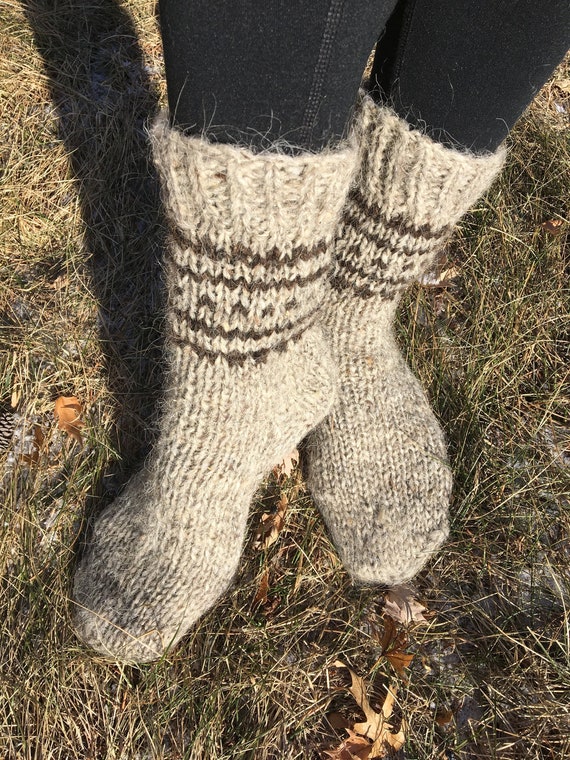This photograph features a pair of knit wool socks, commonly known as salt and pepper or heather style, that are brownish-tan in color with reddish-brown or dark brown bands around the ankles, accented by dots between two rows of stripes. The socks, which rise up to about shin level, are worn over black tights. The person modeling them is standing in dry grass with some scattered leaves, with their right foot pointed to the lower left corner and their left foot more towards the middle right. The image captures the scene outdoors at a low sun angle, casting a shadow towards the back. The thick, woolly socks appear suitable for cold weather, providing warmth and comfort.